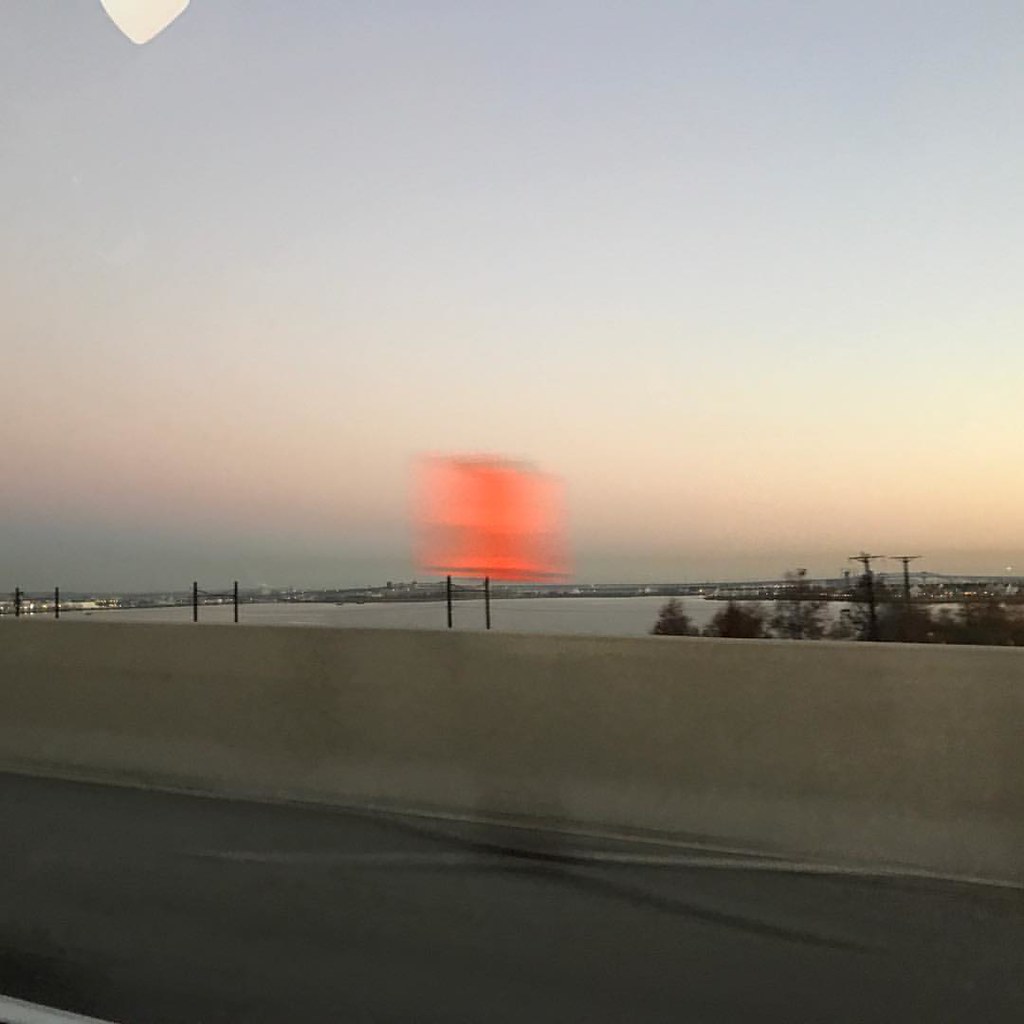This outdoor image captures a scene likely set beside a roadway. In the bottom left corner, a white painted line on a dark gray asphalt surface is clearly visible, indicating the edge of this road. Adjacent to the roadway is a short concrete retaining wall, typical for areas with potential hazards.

In the background, the horizon features an abstract, blurry red area that appears superimposed or reflected. This vivid red smudge, surrounded by gradients of pink, resembles an explosion of color or perhaps a setting sun on an overcast day. The sky above transitions from these pink hues to a gradient of gray and blue.

Below the sky, a serene body of water stretches toward the horizon. Across the water, there is land with discernible buildings, although details are blurred. White areas and structures suggest the presence of homes or neighborhoods, adding to the tranquil yet slightly mysterious ambiance of the scene.